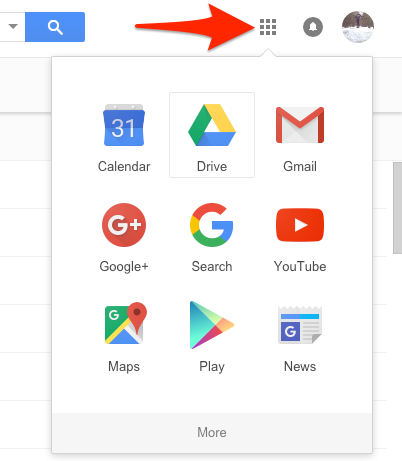The image appears to be a screenshot taken from a digital device, such as a computer, laptop, or smartphone. Featured prominently in the center is a main rectangular frame containing nine distinct application icons, each with its own label. 

1. **Calendar**: The upper left icon depicts a small calendar symbol and is labeled "Calendar."
2. **Drive**: Adjacent to the Calendar icon is one with a triangular design in yellow, green, and blue hues, labeled "Drive."
3. **Gmail**: Next is an envelope icon featuring a red "M" outline, labeled "Gmail."
4. **Google Plus**: Positioned in the next row down is a red circle containing a large "G" with a plus sign (+), labeled "Google Plus."
5. **Search**: Adjacent to Google Plus, there's an icon with a capital "G" in broken sections of red, yellow, green, and blue, labeled "Search."
6. **YouTube**: Following is an icon that resembles an elongated oval with a red background and a white arrow pointing to the right, labeled "YouTube."
7. **Maps**: Next in line is an icon featuring a small square, labeled "Maps."
8. **Play**: Below Maps, there is an icon labeled "Play."
9. **News**: The last icon in this sequence shows a newspaper graphic and is labeled "News."

Each icon is visually distinct, utilizing a combination of colors and shapes to represent different Google applications and services.